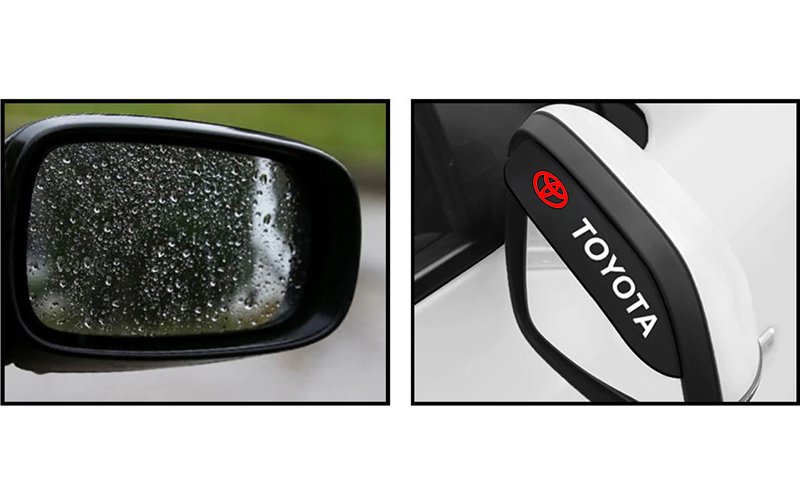In the composite image, two side-by-side photos are outlined in black. The left photo is a close-up shot of a car's black plastic side mirror, beaded with numerous raindrops. A slightly green and gray background suggests an outdoor, possibly rainy, setting. The right photo, against a white background, features another side mirror, but this one is white with a black visor and the Toyota logo printed in red. Below the logo, "Toyota" is written in white letters. This mirror is equipped with a rain shield, designed to protect it from getting wet, and is attached to a white car door. The images, showcasing mostly neutral colors with some red and green accents, appear to be professional advertising shots of car accessories, likely intended for promotional use by Toyota.